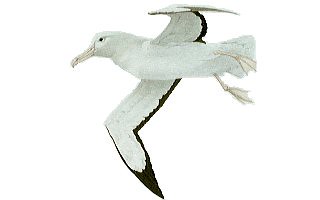The digital artwork features a meticulously detailed depiction of a seagull in flight against a stark white background. The seagull is oriented horizontally, flying from the right to the left side of the image. Its head is turned towards the left, showcasing its long, hooked beak that has a pearly beige hue matching its legs and webbed feet. The seagull's body and outstretched wings are predominantly white, with subtle gray shading adding depth. A striking detail is the black border along the edges and tips of its very long wings, which curve sharply downward towards the end, creating a dynamic sense of motion. The bird’s eyes are black, and its tail, although fanned out, is relatively short compared to its expansive wingspan. The seagull's graceful flight is captured with its head slightly downturned and wings in a flowing, downward arc, bringing a sense of natural elegance to the composition.